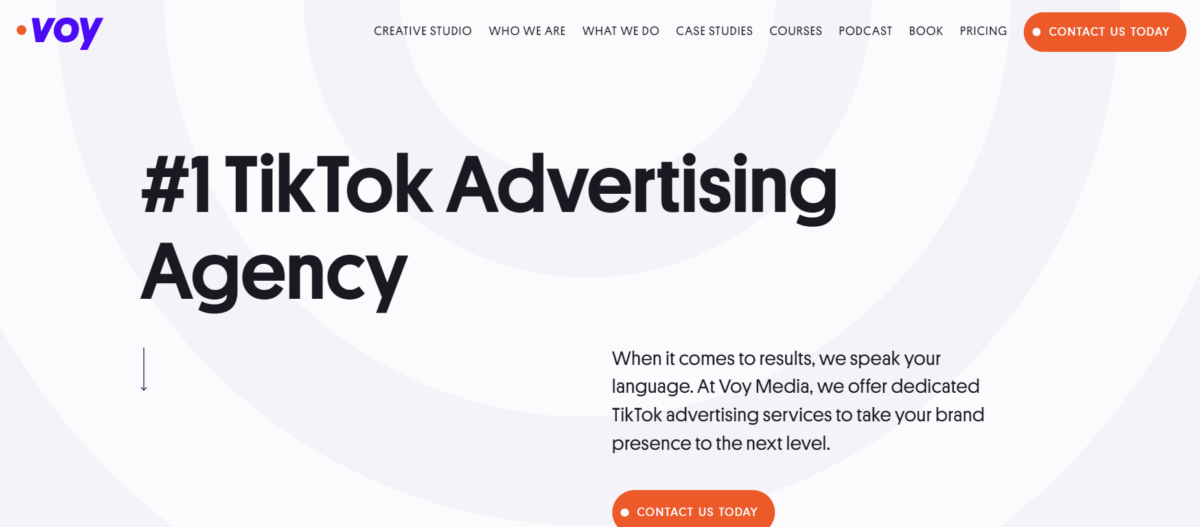Here's a cleaned-up and detailed descriptive caption based on the provided information:

---

A screenshot of a web page for Voy Media, a business branded as a "Creative Studio." The key sections listed on the page include: "Who We Are," "What We Do," "Case Studies," "Courses," "Podcast," "Book," "Pricing," and "Contact Us Today." At the top, there's a bold headline declaring Voy Media as the "#1 TikTok Advertising Agency." Beneath this, in smaller text, it reads, "When it comes to results, we speak your language. At Voy Media, we offer dedicated TikTok advertising services to take your brand presence to the next level." Below this is a prominent red button with white text that says, "Contact Us Today." The overall page design features a white or grayish-white background with black text. The company logo is in blue lowercase letters, "voy."

---